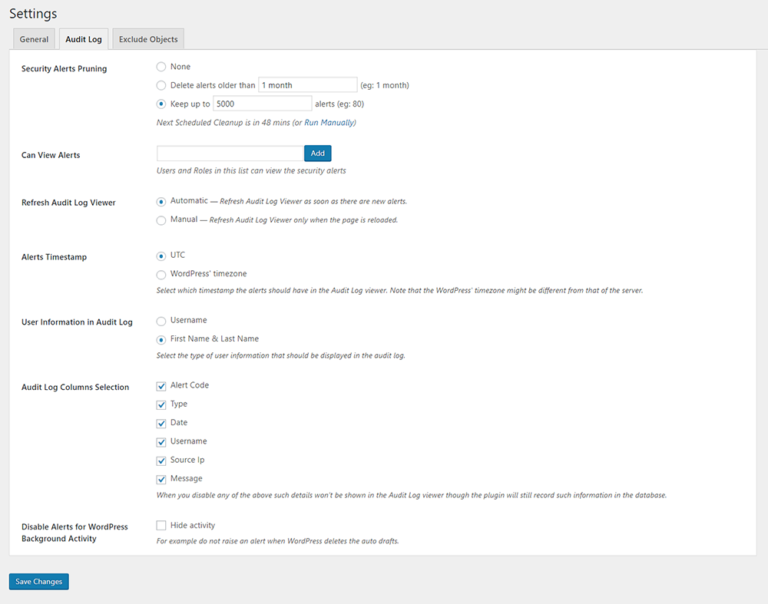The image displays a website’s settings page with a light gray background around the borders. The top of the page features the title "Settings" followed by the category name "General." The "Audit Log" tab is open, with an adjacent tab labeled "Exclude Objects." The main body of the page has a white background and contains several options related to security alerts and audit log settings. 

- The "Security Alerts" section is bold and aligned to the left. 
- Next to "Security Alerts," on the right, it reads "None," with a circular selection icon to the left.
- Another option states "Delete alerts older than one month," with an unselected circle to the left.
- Below is a section with a selected circle marked "Keep up to" and an input box containing "5,000 alerts."

Further down:
- The option "Can view alerts" appears on the left with a rectangular input box beside it and an "Add" button to the right.
- "Refresh audit log viewer" is listed beneath that.
- Below this, there are labels for "Alerts time stamp," "User information," and "Audit log."
- The "Audit log column section" follows, with all its options checked.
- At the bottom of this section is the option to "Disable alerts for WordPress background activity," with checkboxes for selection on either side.

The bottom of the page features a "Save Changes" button aligned to the left, with a blue background.